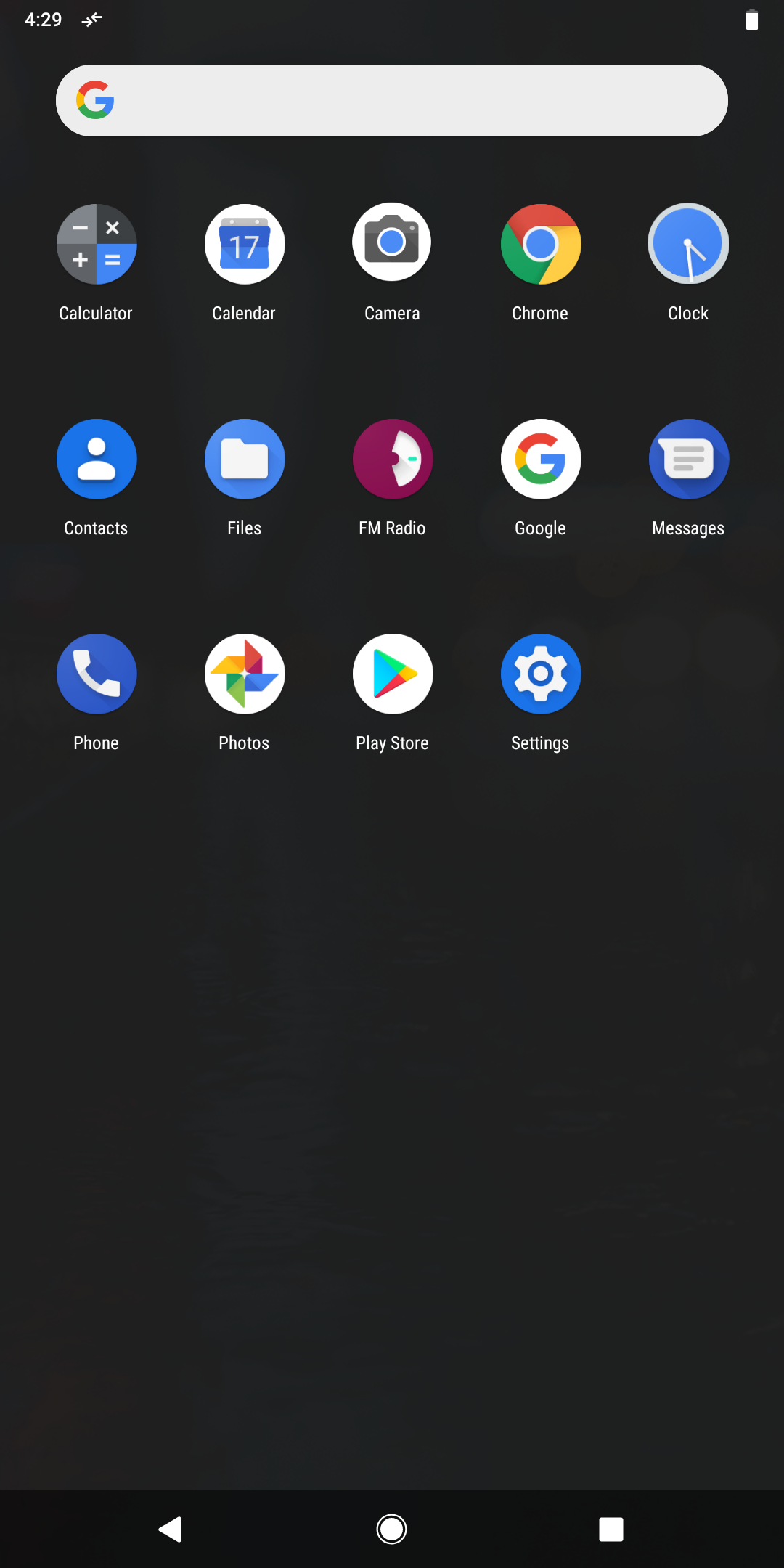The image depicts a screenshot of a smartphone's home screen with a black wallpaper. In the upper left corner, the time is displayed as "4:29." The time is ambiguous as it doesn't indicate whether it's a.m. or p.m. Adjacent to the time is a symbol of two arrows facing each other closely, the meaning of which is not immediately recognizable. On the right side of the screen, the battery icon is predominantly white, suggesting a high charge level.

Just below this status bar, there is a light gray oval featuring the Google "G" logo, which is composed of four colors: red at the top, followed by yellow, green, and blue. Below this search bar, the screen is organized into three rows of app icons, each labeled with their functions in white text:

- **First Row:** Calculator, Calendar, Camera, Chrome, Clock.
- **Second Row:** Contacts, Files, FM Radio, Google, Messages.
- **Third Row:** Phone, Photos, Play Store, Settings.

Each icon exhibits a distinct color scheme, predominantly featuring blue backgrounds with white and gray elements:
- The **Clock** icon has a blue background with a white and gray outline.
- **Contacts** shows a blue background with the white silhouette of a person.
- **Files** features a blue background with a white folder icon.
- **Messages** has a blue background with a white and gray text message icon.
- **Phone** displays a blue background with a white telephone receiver.
- **Settings** is represented by a blue background with a white gear.

Additionally, the **Calendar** app has a white background featuring a blue box with the number "17" in gray. The **Calculator** icon is divided into four quadrants representing different operations: subtraction, multiplication, addition, and an equal sign in blue located in the lower right-hand corner.

This detailed description captures the overall layout and appearance of the smartphone's home screen, highlighting the colors, symbols, and arrangement of various app icons.